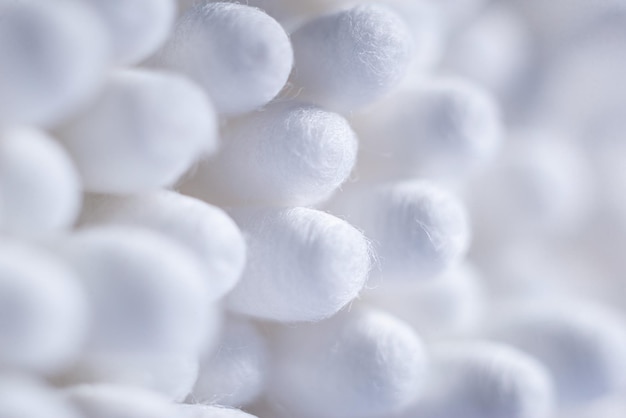The image is a highly detailed, close-up shot of numerous Q-tip heads clustered together. The primary focus is on three or four Q-tips in the center, revealing the fine texture of the soft cotton tips in intricate detail. The cluster includes at least 16 to 17 Q-tips, although it's challenging to count the exact number due to the surrounding blur, which obscures the edges. The overall color of the image is predominantly white with slight shadowing, suggesting the light source is positioned in the upper right-hand corner, casting gentle shadows that add depth and dimension to the composition. The sharp focus in the center gradually transitions to a blur towards the periphery, emphasizing the central grouping in crisp clarity.